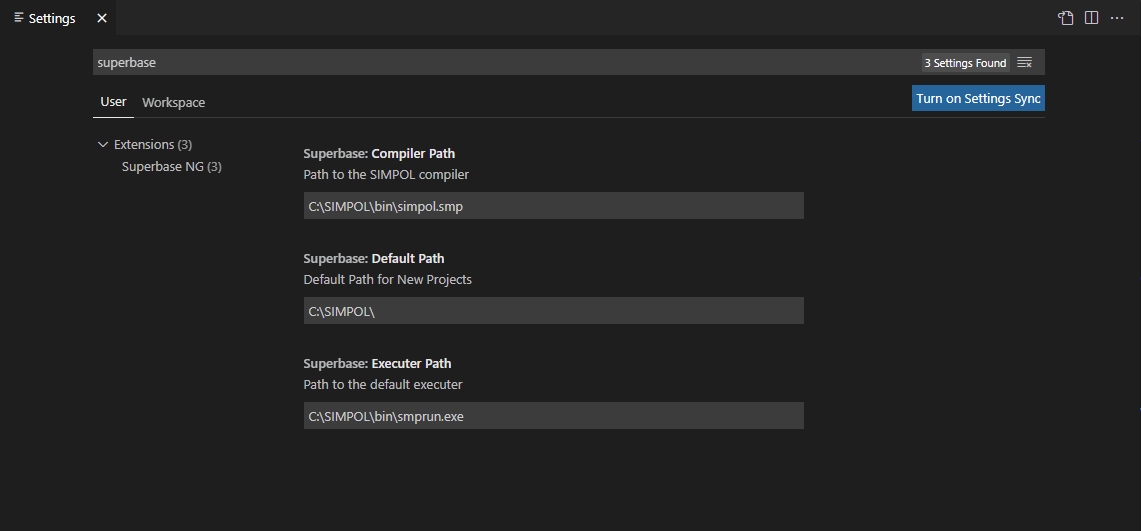The image depicts an interface screen with a predominantly black background. In the upper left corner, there's a "Settings" label accompanied by a close (X) icon. The upper right corner features several icons: one depicting a page with a corner turned down and an arrow, another illustrating a page with a horizontal line, and a trio of vertical dots.

Below, there is a gray field with the label "SuperBase." Adjacent to this, a notification states "Three settings found," followed by an icon of four horizontal lines stacked together, ending in a close (X) icon in the bottom right of this segment.

Further down, the interface lists multiple settings: the "User" section, highlighted, followed by "Extensions," noting three items, "SuperBase NG," also with three items, and a "SuperBase Compiler Path" entry, which specifies the path to the SIMPOL compiler: `C:\SIMPOL\bin\SIMPOL.SMP`. Directly below, the "SuperBase Default Path" entry indicates the default location for new projects: `C:\SIMPOL\`.

Lastly, the "SuperBase Executor Path" setting identifies the path to the default executor: `C:\SIMPOL\bin\SIMPOL.SMPRUN.EXE`.